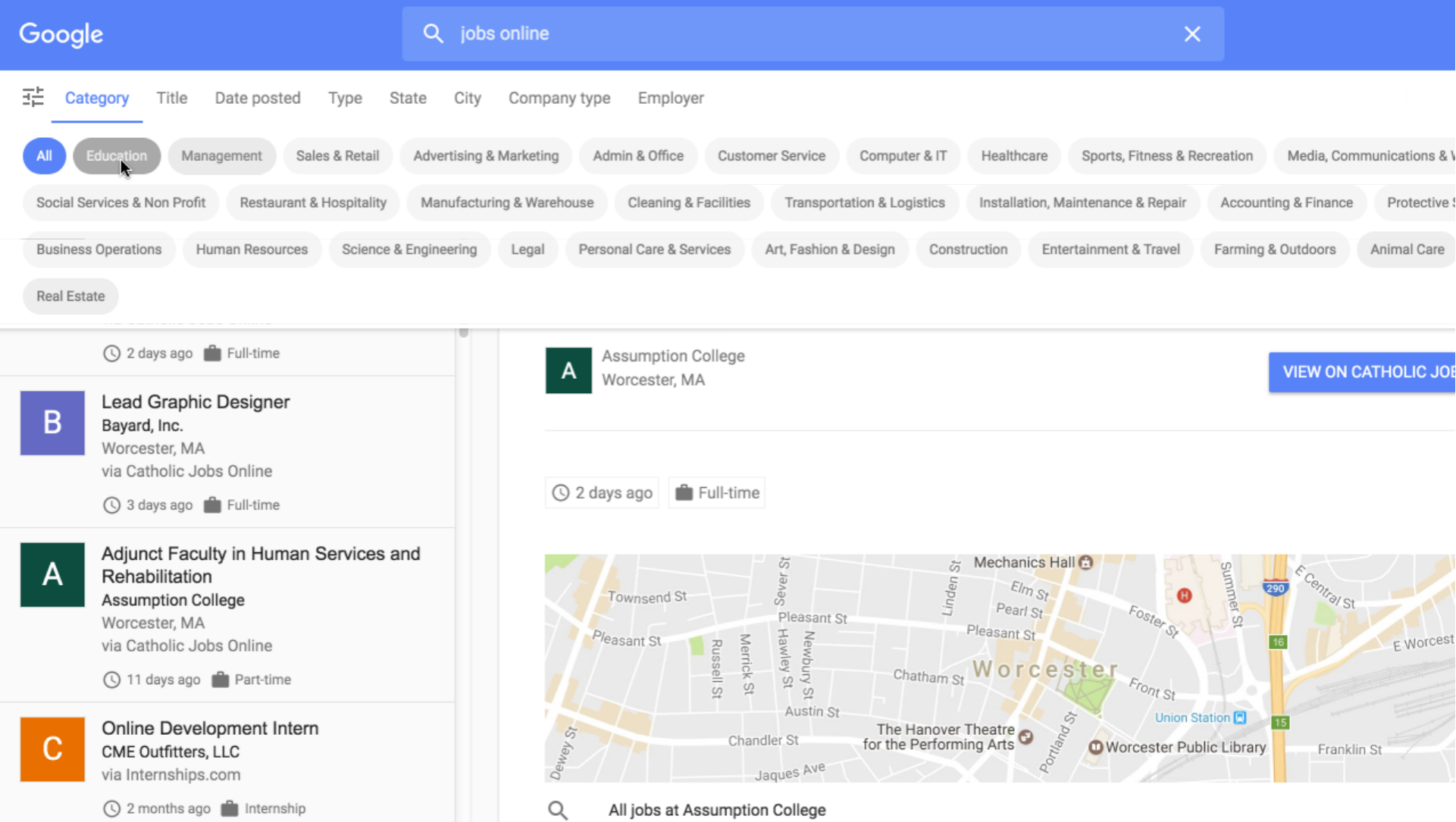The image depicts a Google search results page for online job listings with multiple categories including job title, date posted, job type, location (state and city), company type, and employer. A highlighted result shows a full-time job at Assumption College in Worcester, Massachusetts, posted two days ago, with a blue button offering an option to view the job on Catholic Jobs. A map indicating directions to Assumption College and a specialized search bar for all jobs at Assumption College are also visible. On the left side, additional listings include: a full-time Lead Graphic Designer position at Bayard Incorporated in Worcester, Massachusetts, posted three days ago on Catholic Jobs; a part-time Adjunct Faculty position in Human Services and Rehabilitation at Assumption College, Worcester, Massachusetts, posted 11 days ago on Catholic Jobs; and an internship position for an Online Development Intern at CME Outfitters LLC from Internships.com, posted two months ago.